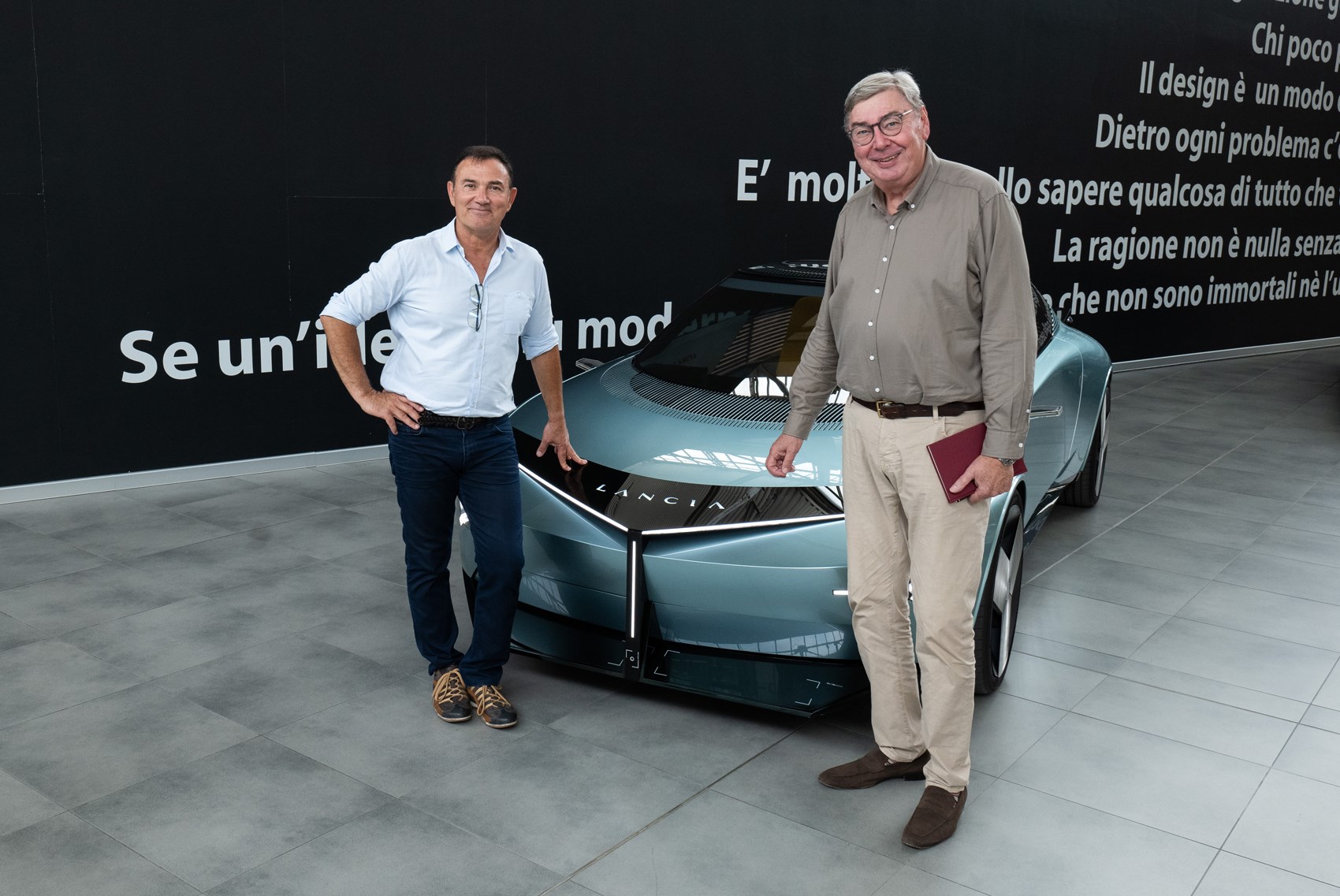The photograph showcases two gentlemen standing proudly in front of a sleek, light blue Lancia sports car at a showroom or exhibition event. The backdrop features a black wall adorned with various textual details in Italian. The man on the right is in his 50s, dressed in a white button-down shirt with glasses tucked into the buttons, dark denim jeans, and brown shoes with light brown laces. He stands with his hand on his hip, smiling warmly at the camera. Next to him, the taller, older gentleman, possibly in his 60s or 70s, has white hair and is also smiling. He wears a brown button-down shirt, khakis, a brown belt, and brown shoes, and holds a red notebook in his left hand. Both men exude a casual elegance, enhancing the professional ambiance of the photo.